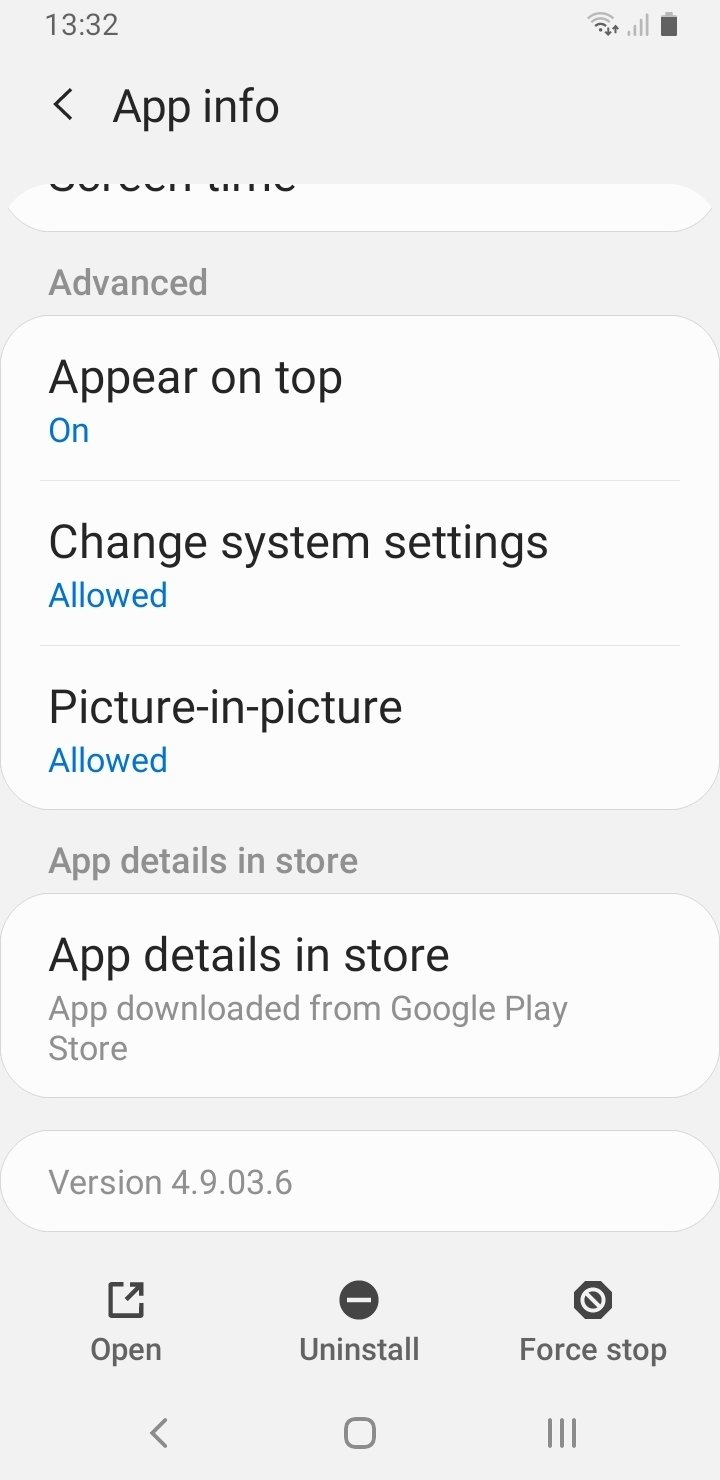**Detailed Caption:**

The image appears to be a screenshot of the settings section within an Android device. The time displayed in the upper left corner is in military format, reading 13:32. On the upper right corner, a full Wi-Fi signal icon is visible next to a less than full cellular signal bar. The battery icon shows nearly full capacity, approximately 90%.

Beneath the status bar, on the left side, there’s an arrow pointing to the left followed by the label "App info." Partially visible below this, a rounded box appears to be cut off, with some incomplete text. Further down, the text "Advanced" is clearly visible. Next, a highlighted blue box indicates the option labeled "Appear on top" is switched 'On.'

The next section, titled "Change system settings," has an "Allow" option beneath it, signified by a separator line before the next heading, "Picture." This section also contains an "Allow" option highlighted in blue. Below this, the text "App details in store" is shown in gray font.

Near the bottom of the screen, within a rounded rectangle, the label "App details in store" appears again, signifying that the app was downloaded from the Google Play Store. Additional information includes the app version, and three icons are displayed at the bottom of the screen.